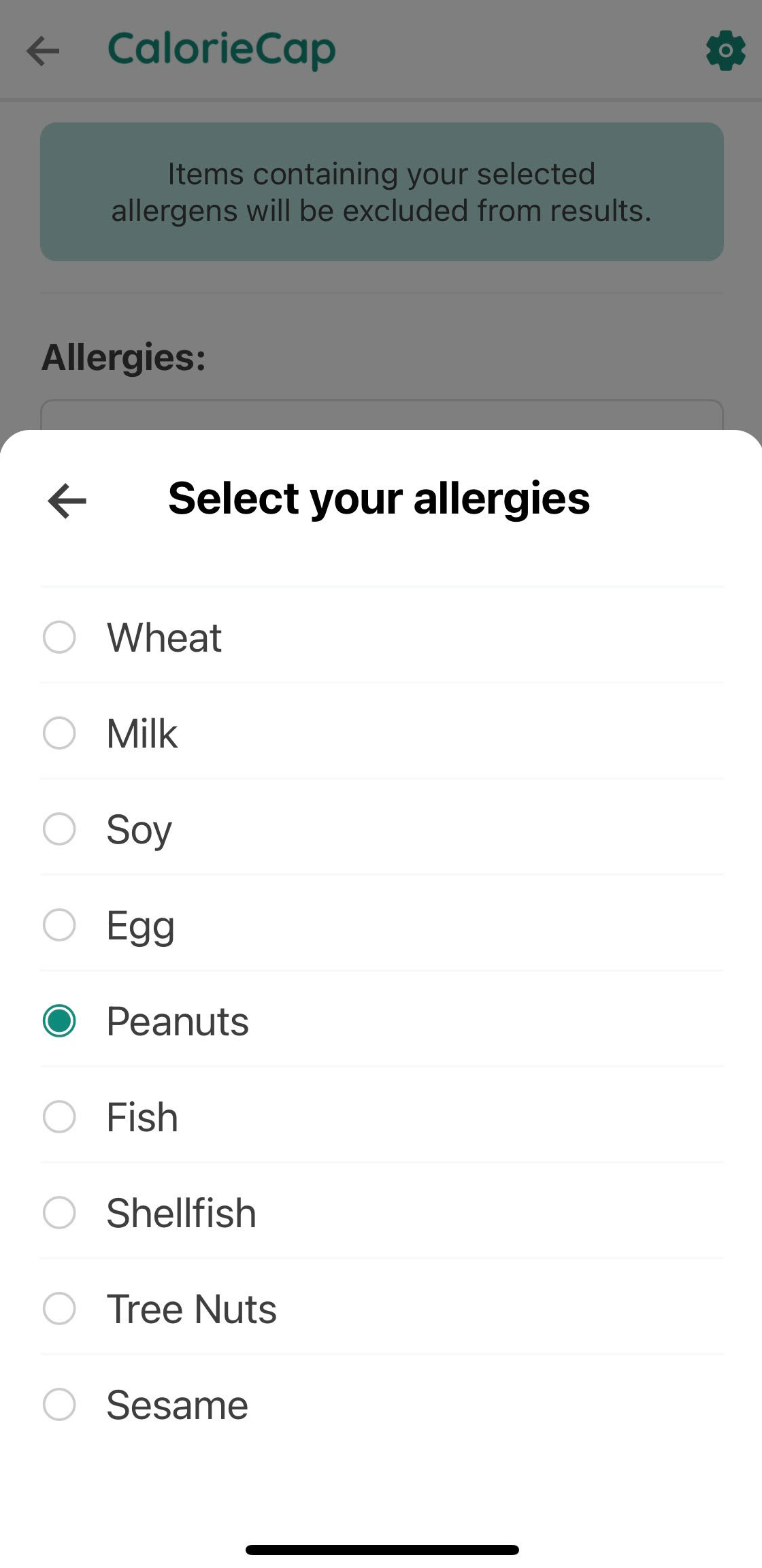**Detailed Caption:**

The image showcases a feature in the 'Calorie Cap' app designed for users with specific dietary restrictions. At the top, there is a green arrow pointing to the left, accompanied by a settings icon on the right. The text, slightly blacked-out for a drop-down page, reads, "Calorie Cap." Below, a message in clear text states, "Items containing your selected allergens will be excluded from results." This is followed by a drop-down menu labeled "Select your allergies" set against a black and white background. 

In this menu, users can select from a list of common allergens, each with a clickable dot to indicate their choice. These allergens include wheat, milk, soy, egg, peanuts, fish, shellfish, tree nuts, and sesame. The highlighted option shows the dot next to "peanuts" circled in green, indicating that this allergen is selected to be excluded from search results.

This visual representation emphasizes the app’s filter functionality, simplifying the process of avoiding allergens. Users can effortlessly ensure that any food items containing peanuts, for instance, are excluded from their search results, enabling safer food choices without the need for manual checks.